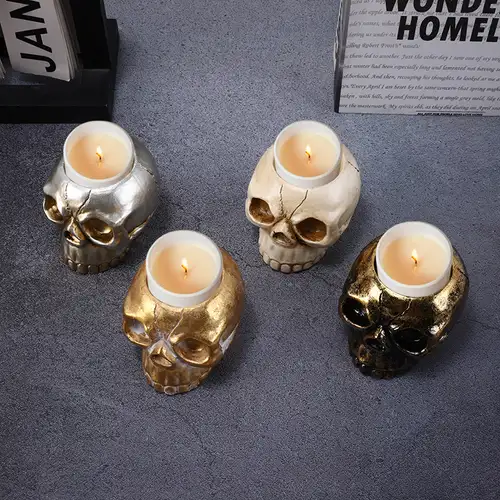This is an overhead photo featuring four skull-shaped candle holders, arranged in a row on a dark grey to blue surface with visible cracks. From left to right, the skulls are: silver with gold eyes, all gold, bone-colored, and a dark gold or nearly charcoal hue. Each skull holds a small white votive candle with a ridged edge, all of which are lit, casting a neutral and somewhat dark tone to the image. In the far left corner, there is a partial view of an item with the word 'January,' adding a subtle context to the scene.